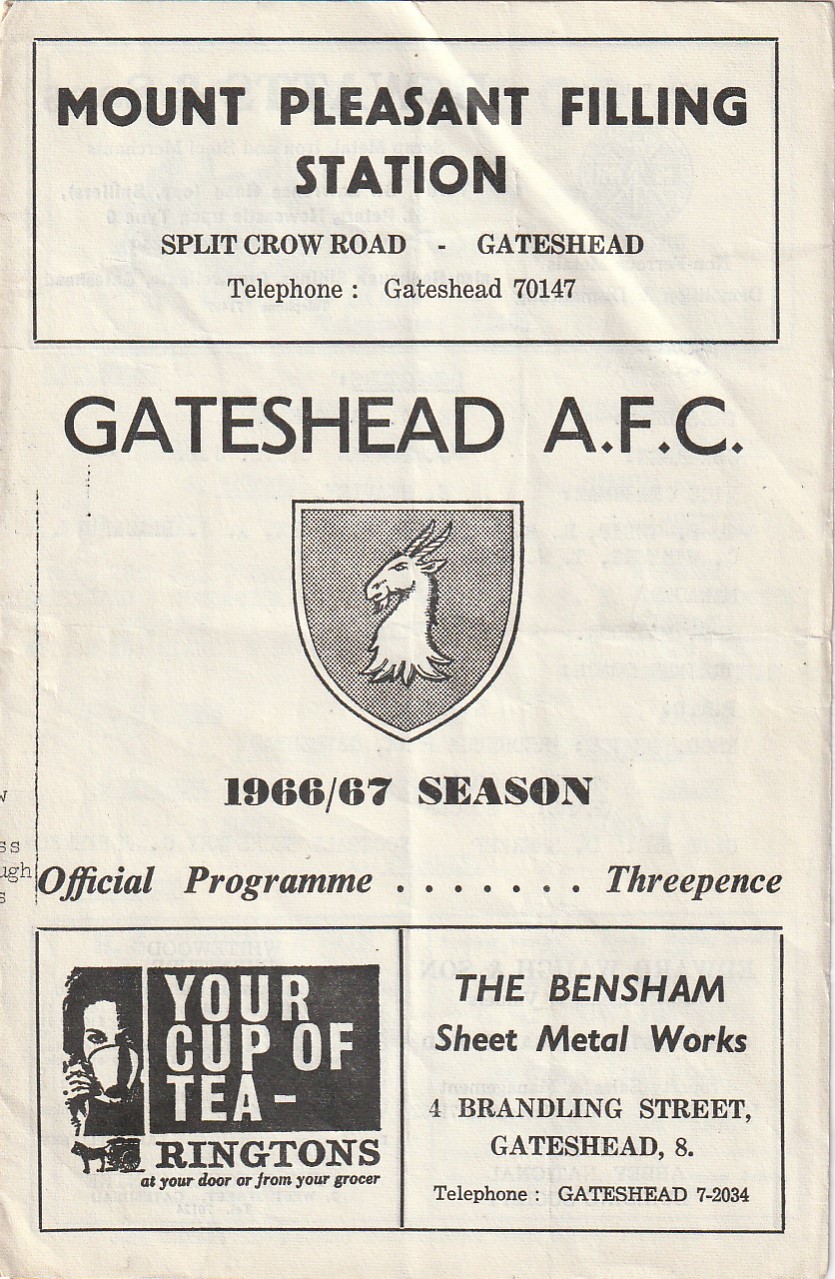The image appears to be an old, creased, and worn official program for a match day of Gateshead AFC from the 1966-67 season, printed in black and white. At the top, there is an advertisement for Mount Pleasant Filling Station located at Split Crow Road, Gateshead, with the contact number Telephone Gateshead 70147. Below that, in bold block capitals, it reads Gateshead AFC followed by a crest featuring what looks like a goat's head as part of the logo. The program is marked with "Official Programme" and "three pence." At the bottom left, there is an advertisement for Ringtons, depicting a woman sipping a cup of tea, and the text reads, "Your Cup of Tea, Ringtons At Your Door, or From Your Grocer." On the bottom right, there is another advertisement for the Bensham Sheet Metal Works, detailing the address as Bradling Street, Gateshead 8, and the contact number Telephone Gateshead 7-2034. The overall layout and presentation suggest it was possibly taken from a newspaper or a similar publication.